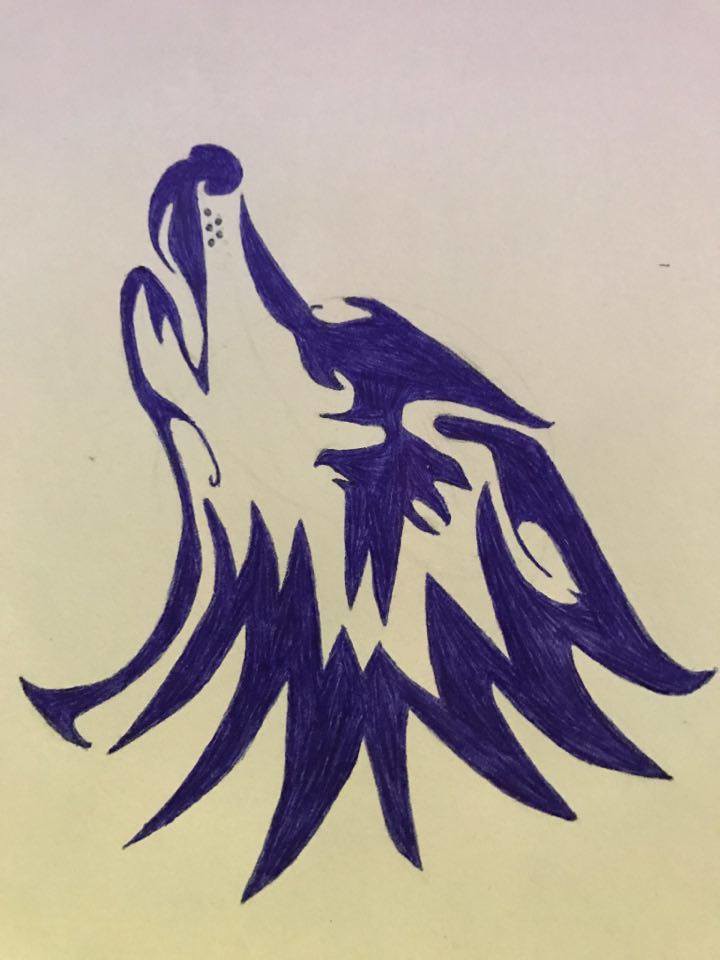A detailed artwork showcases a howling wolf, meticulously rendered in deep blue and white hues. The striking contrast between these two colors vividly depicts the textured fur, defined nose, and delicate whiskers of the wolf. Positioned against a pale background, the wolf’s head is prominently outlined, with its nose pointed skyward and mouth open in a powerful howl. The closed eyes of the wolf emphasize the intensity and emotion of the moment, capturing a timeless gesture of nature in an elegant and minimalist composition.